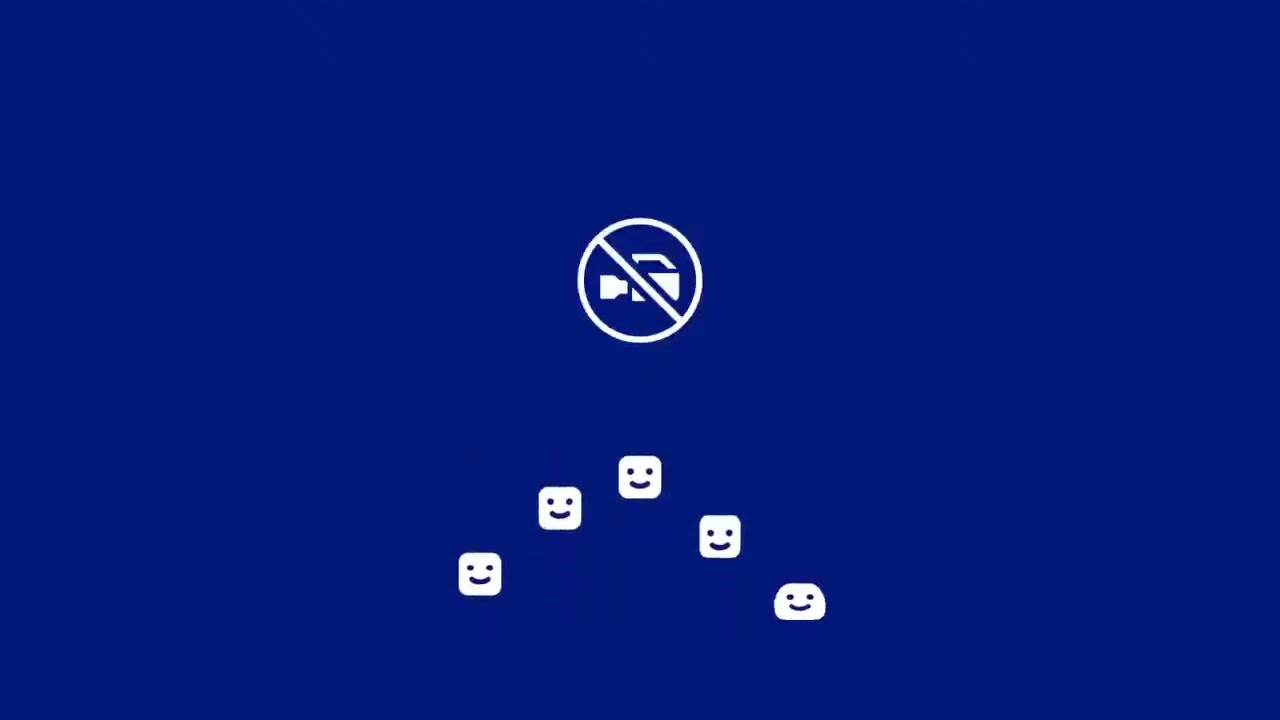The image is a color illustration in blue and white, presented in a landscape orientation. Dominating the center, toward the top, is a prominent white circle with a diagonal slash through it, overlaying the outline of a video camera, signifying no recording. Below this circle are five white, square-shaped smiley face emojis arranged in a triangular formation, set against the entirely blue background. Notably, the smiley face at the bottom right is slightly flattened compared to the others. The image's graphic art style is reminiscent of a movie theater lobby sign or a brochure requesting visitors not to film.